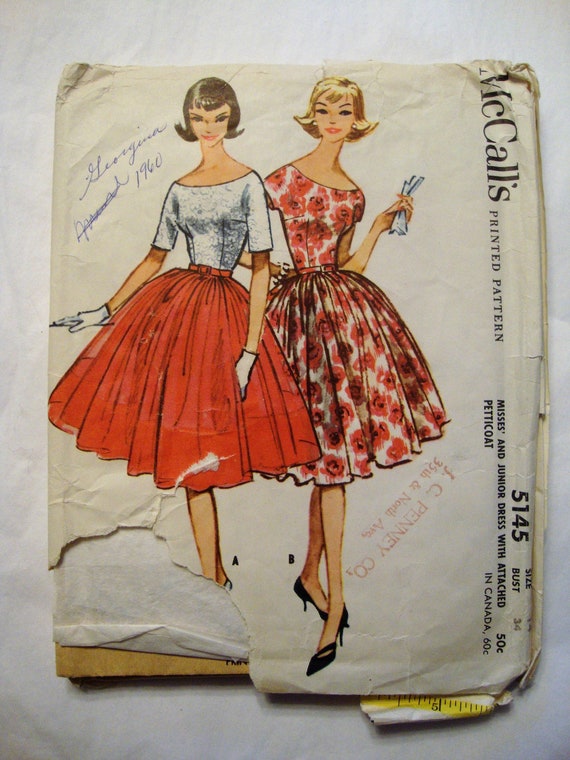The image shows a McCall's printed pattern envelope titled "Mrs. and Junior Dress with Attached Petticoat," labeled with pattern number 5145, priced at 50 cents in the U.S. and 60 cents in Canada. The envelope features a cartoon image of two women; the woman on the left wears a white top paired with a red skirt, and the woman on the right dons a white gown adorned with red floral patterns. Notably, the design is autographed by someone named Georgina, dating back to 1960, and there's a crossed-out section. The envelope itself is set against a white background, and a yellow measuring tape marked with the number 5 lies at the bottom of the image. The pattern was produced by JCPenney, specifically at the location 35th and North Avenue.